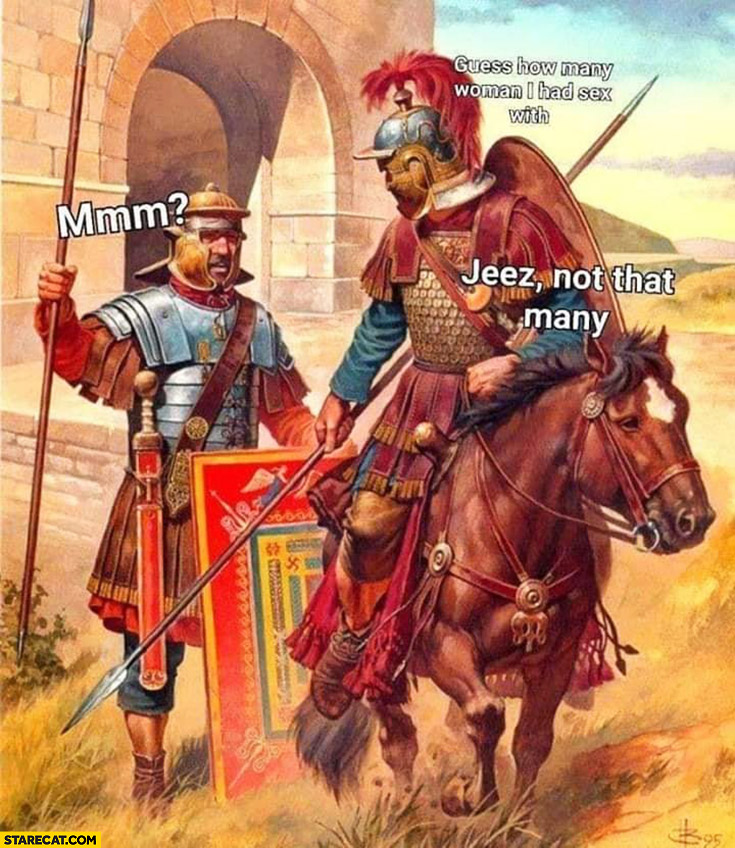In a vividly detailed color illustration reminiscent of historical artwork, two armored men appear poised for battle in a medieval setting. Both men clutch spears, their attire a mix of leather and metal in hues of gray, brown, and red. The man on the left stands firmly on the ground, his armor reflecting an Asian style and a shield painted red, yellow, and blue at his side. His expression is marked with a text bubble saying "MM?" The right side of the image features a man atop a small brown horse with a distinctive white patch on its forehead. The horse, outfitted in a brown leather harness, lifts one front leg as if mid-step. This rider wears a metal hat adorned with a striking red feather and gazes back over his right shoulder toward his comrade. Above him, white text reads, "Guess how many women I had sex with?" with a follow-up caption below him stating, "Geez, not that many." They stand before a stone building with an open arch, and in the background rolls a hilly, grassy landscape under a vast sky. The overall setting evokes times long past, perhaps hundreds of years ago, and the layout suggests a scene from a meme.